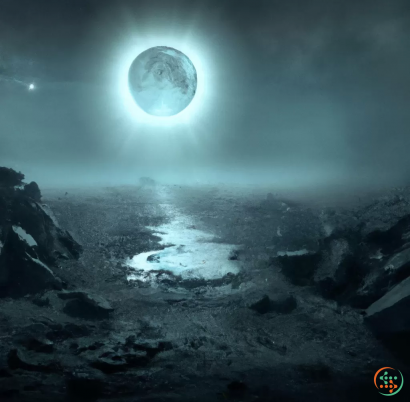The image is a digital drawing, presented in a perfectly square format, approximately 3 inches by 3 inches. The top half of the background features a greenish-black sky with an eclipse-like phenomenon: a large, circular celestial body—possibly a moon or planet—shines with a bright, white halo that starbursts outward. This celestial body is depicted in shades of blue and gray, and it casts a blue-gray hue over the entire scene.

Below the hauntingly illuminated sky, the bottom half of the image reveals a stark, rocky terrain. The dark, black, and gray landscape is characterized by rugged alcoves and a central valley that hosts a small pool of water, suggesting a dried-up stream might have once fed it. 

In the lower right-hand corner of the image, a distinctive circular element is outlined: the left half in red and the right half in green. Within this circle, a green arrow points to the left, overlapping a red arrow pointing to the right. This design element stands out against the otherwise somber and mysterious landscape, adding an intriguing focal point to the lower corner of the dark, evocative scene.